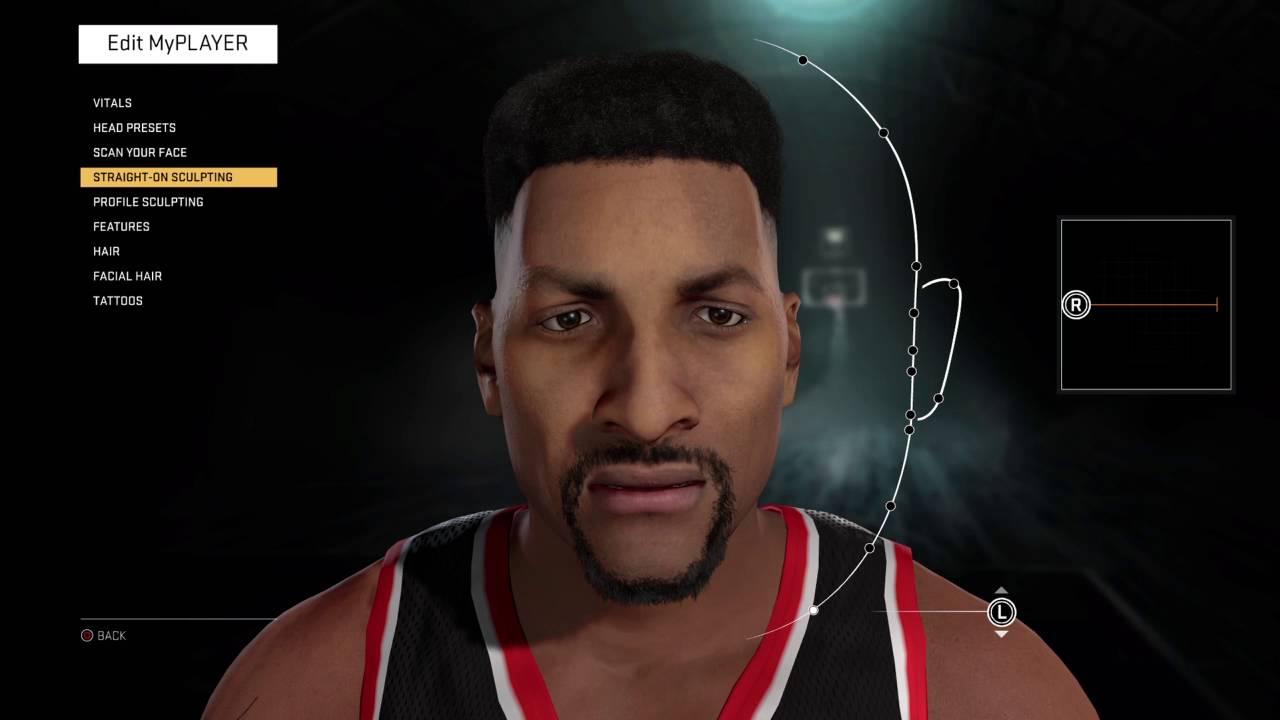This is a detailed screenshot from a video game player's customizer interface. In the top left corner, there's a prominent white rectangular button labeled "Edit My Player." Below this, a vertical list of options is displayed, each on a separate row. The options are: "Vitals," "Head Presets," "Scan Your Face," "Straight-On Sculpting," "Profile Sculpting," "Features," "Hair," "Facial Hair," and "Tattoos." Among these, "Straight-On Sculpting" stands out with its yellow highlight, indicating it is the currently selected option, while the rest are displayed in white text.

To the right of this menu is a visual of a customizable character. The character depicted is a black male with short hair and a goatee beard. He is dressed in a black jersey, and the view captures him from the top of his head down to his shoulders. This setting provides a detailed and interactive environment for players to personalize their in-game avatars meticulously.